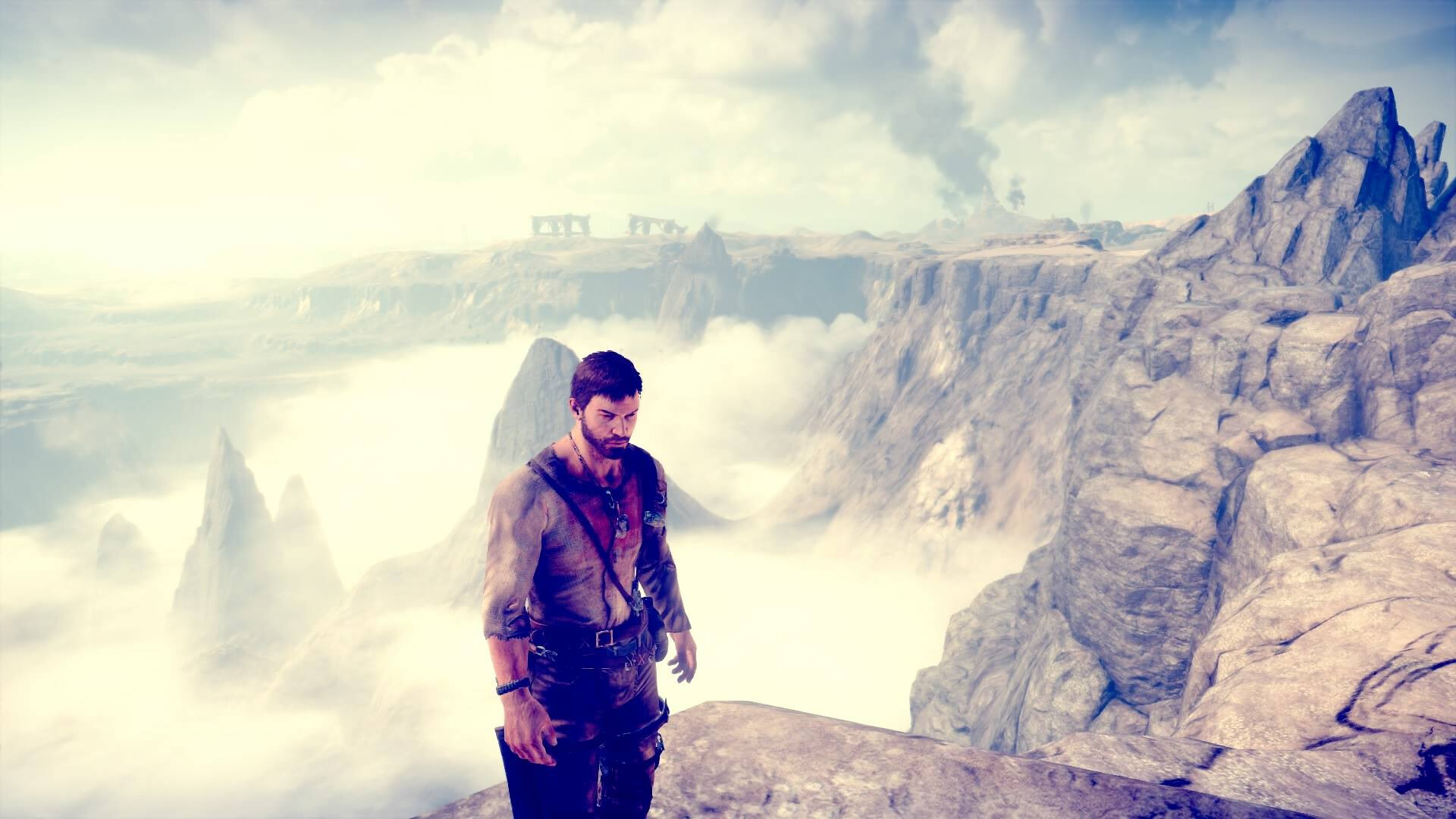In this striking image, which appears to be either a screenshot from a game or a piece of intricate artwork, the focal point is a man standing composedly. His stance suggests a sense of readiness and contemplation as he gazes at a 45-degree angle away from the viewer. He has cropped brown hair and a short, rugged beard that adds to his adventurous appearance. He is wearing a light-colored shirt, possibly white or gray, with one sleeve casually rolled up to his forearm while the other remains unrolled. Complementing his shirt are his brown pants, rugged and practical for the terrain. Draped over his shoulder is a satchel, hinting at a long journey or quest. The man stands at the pinnacle of a cliff, immersed within an expansive mountain range. Below him, the majestic peaks pierce through the clouds, creating a sublime and ethereal atmosphere that underscores the grandeur of his vantage point.